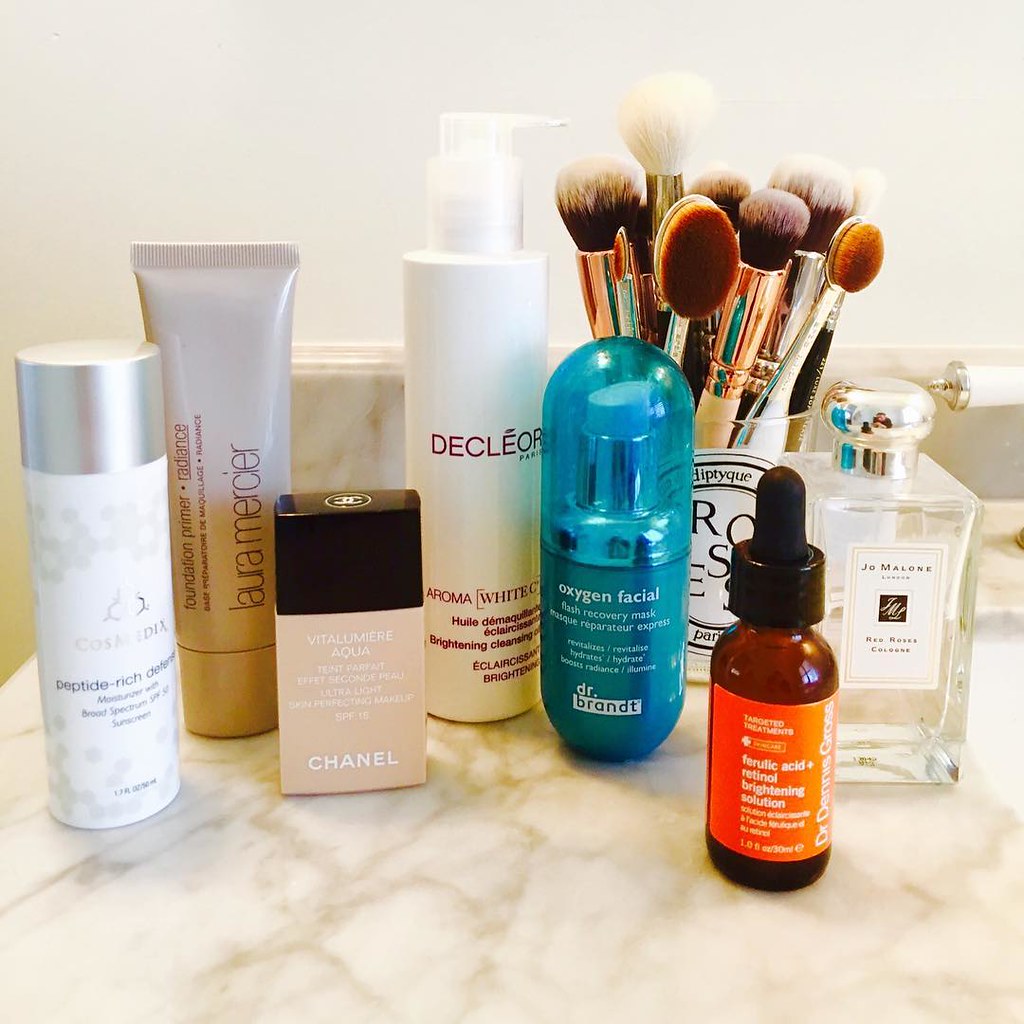The image presents a neatly arranged countertop scene, viewed from above. The countertop occupies the lower section of the image and features an off-white surface with a subtle, medium brown marble pattern. The upper section showcases a plain off-white back wall, providing a neutral backdrop that allows the items on the counter to stand out. 

Central to the scene are several meticulously placed skincare and makeup products. On the far left sits a white canister with a sleek silver top, labeled "Peptide Rich," though the subsequent text is indistinguishable. Adjacent to this is a light brown tube, slightly taller in stature, branded with "Laura Mercier" along its side. 

Moving further to the right, there's a rectangular container with a contrasting black top and a cream-colored base, suggesting it might be a spray or pump-style product. Completing the arrangement is a cup brimming with makeup brushes and an item resembling a perfume bottle. The careful placement and variety of the products imply an intentional display, perhaps highlighting a daily skincare or makeup routine.